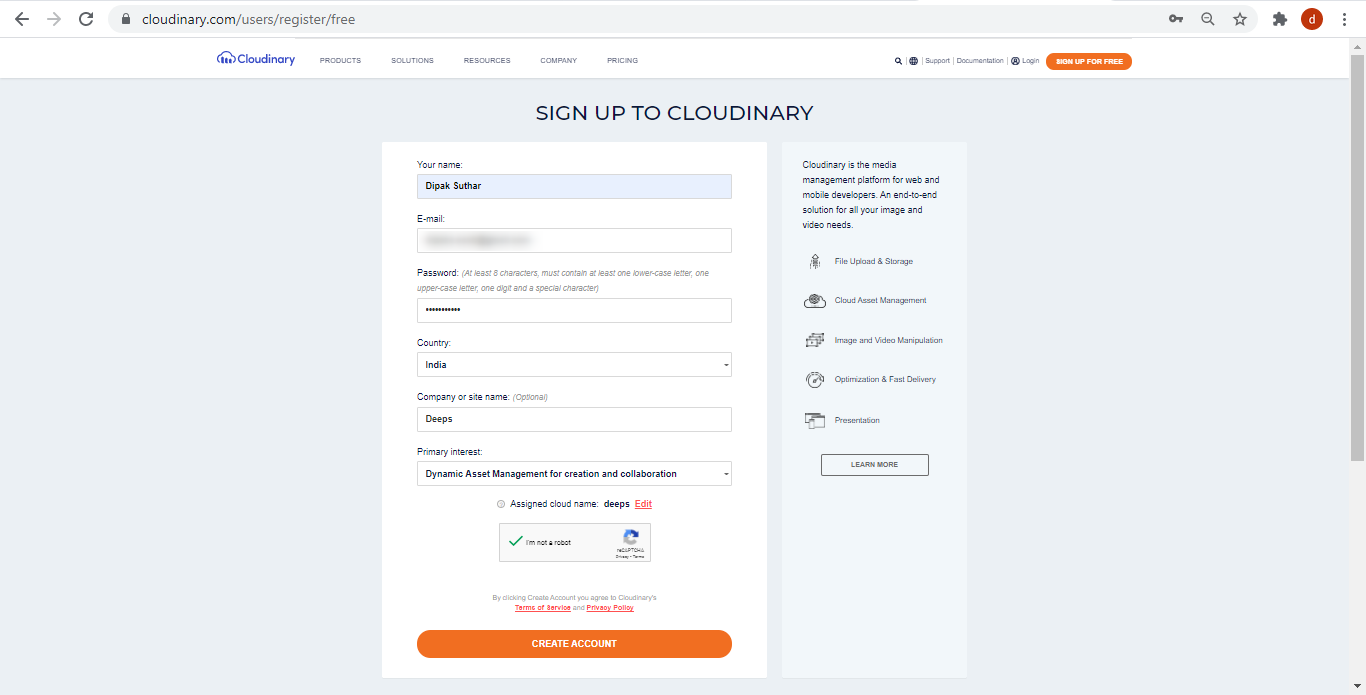A detailed screenshot description of the Cloudinary registration webpage:

The screenshot depicts the Cloudinary registration webpage with various elements and features clearly highlighted. At the very top of the browser window, standard navigation buttons are visible, including the back, forward, and reload buttons. The web address bar displays "cloudinary.com/users/register/free," with a padlock icon indicating a secure connection. To the right of the address bar, there are icons for a key, a star (likely for bookmarking), a search icon, a puzzle piece (extensions or plugins), a red circle with a "D" (representing the username’s initial), and vertical three dots for additional options.

Directly below the browser tools, there is a grey navigation bar featuring the Cloudinary logo and the name in blue, followed by small text links for "Products," "Solutions," "Resources," "Company," and likely "Pricing." On the far right of this grey bar, further small text links for "Search Support," "Documentation," and "Login" can be seen. An orange box with white text prominently offers the option to "Sign Up for Free."

Beneath this navigation bar, the background color shifts to a slightly darker grey. Centered in this section is the text "Sign up for Cloudinary." Below this headline are the registration fields. The form begins with the field for "Your Name," pre-filled with "Deepak Sutar." Following this is a field for the email address, which is blanked out for privacy. Next is the password field, accompanied by guidance text specifying that the password must be at least 18 characters long and include one lowercase letter, one uppercase letter, one digit, and one special character. The inserted password is obscured by dots.

Additional fields include "Country," pre-selected as India, "Company or Site Name," which is optional and currently listed as "Deeps," and "Primary Interest," chosen as "Dynamic Asset Management for Creation and Collaboration." The assigned cloud name is "Deeps," which can be edited. A Captcha box confirms the user is not a robot with a checkmark.

At the bottom of the form, a disclaimer states that by clicking "Create Account," the user agrees to Cloudinary's terms of service and privacy policy. The form concludes with a prominent wide orange button labeled "Create Account." 

Adjacent to this button is a grey rectangle containing black text, which explains Cloudinary as a media management platform tailored for web and mobile developers, providing an end-to-end solution for all image and video needs. Icons with descriptions include "File upload and storage," "Cloud asset management," "Image and video manipulation," "Optimization," "Fast delivery," and "Presentation." The segment concludes with a "Learn More" button.